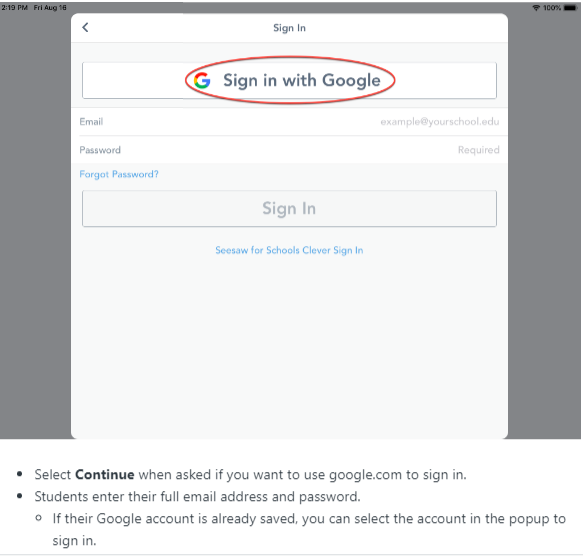Screenshot of a Sign-In Page: 

The image displays a sign-in interface that pops up over a blurred background. At the top of the pop-up box, the text "Sign In" is prominently displayed. Below this header is a large rectangular white box with the Google logo and the text "Sign in with Google." Beneath this option are input fields labeled "Email" and "Password" for manual sign-in. 

If the user has forgotten their password, there's a clickable "Forgot Password?" link for recovery. Towards the bottom of the pop-up, additional instructions and options are provided. The text reads:

- "See CSAW for schools clever sign-in."
- A subsequent instruction points out: "Select 'Continue' and ask if you want to use Google.com to sign in students. Enter their full email address and password."
  - A sub-bullet notes: "If their Google account is already saved, you can select the account in the pop-up to sign in."

Also visible in the pop-up is a mouse icon, symbolizing user interaction. The overall layout is user-friendly, guiding the user through the sign-in process with clear options and instructions.